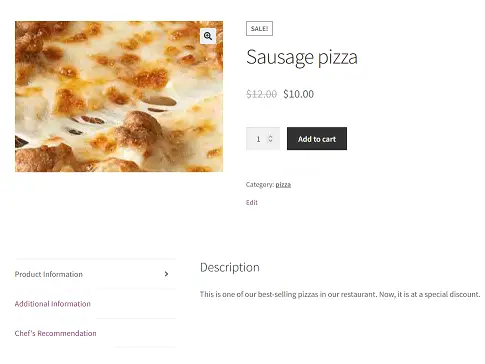Here is a detailed and cleaned-up caption for the image:

---

**Screenshot of Sausage Pizza on Sale**

This screenshot showcases a mouth-watering sausage pizza, generously topped with both large and small pieces of light brown sausage and melted white mozzarella cheese. The pizza, one of the top sellers at the featured restaurant, is now available at a special discounted price of $10, down from the regular price of $12. 

The interface includes a prominent "Add to Cart" button in black and white, as well as an option to edit the order. The section is categorized under "Pizza" and includes several interactive buttons for further information—'Product Information,' 'Additional Information,' and 'Chef's Recommendation.' All text is rendered in a clear black font, ensuring readability.

---